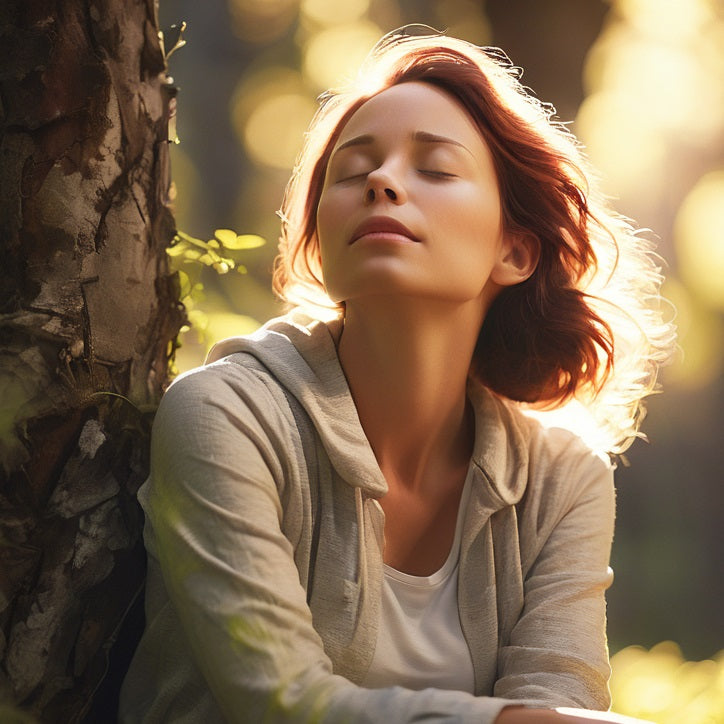This AI-generated image portrays a striking red-haired woman standing outside in a summer woodland setting, leaning against a majestic tree. Her hair, radiant and luxurious, captures the sunlight, creating an ethereal halo with hints of blonde. The woman, with smooth and perfect skin, has her eyes closed, as she slightly tilts her face upward towards the sky, basking in the sun's warm glow. She is dressed in a casual gray zip-up hoodie over a white t-shirt, accented by some yellow spots on her right arm. The tree beside her, detailed with peeling bark in shades of brown and tan, and small green leaves sprouting from its stems, supports her relaxed stance. The background, a blur of vibrant yellows and browns with hints of greenery, further enhances the dreamlike quality of this digitally crafted, close-up scene.